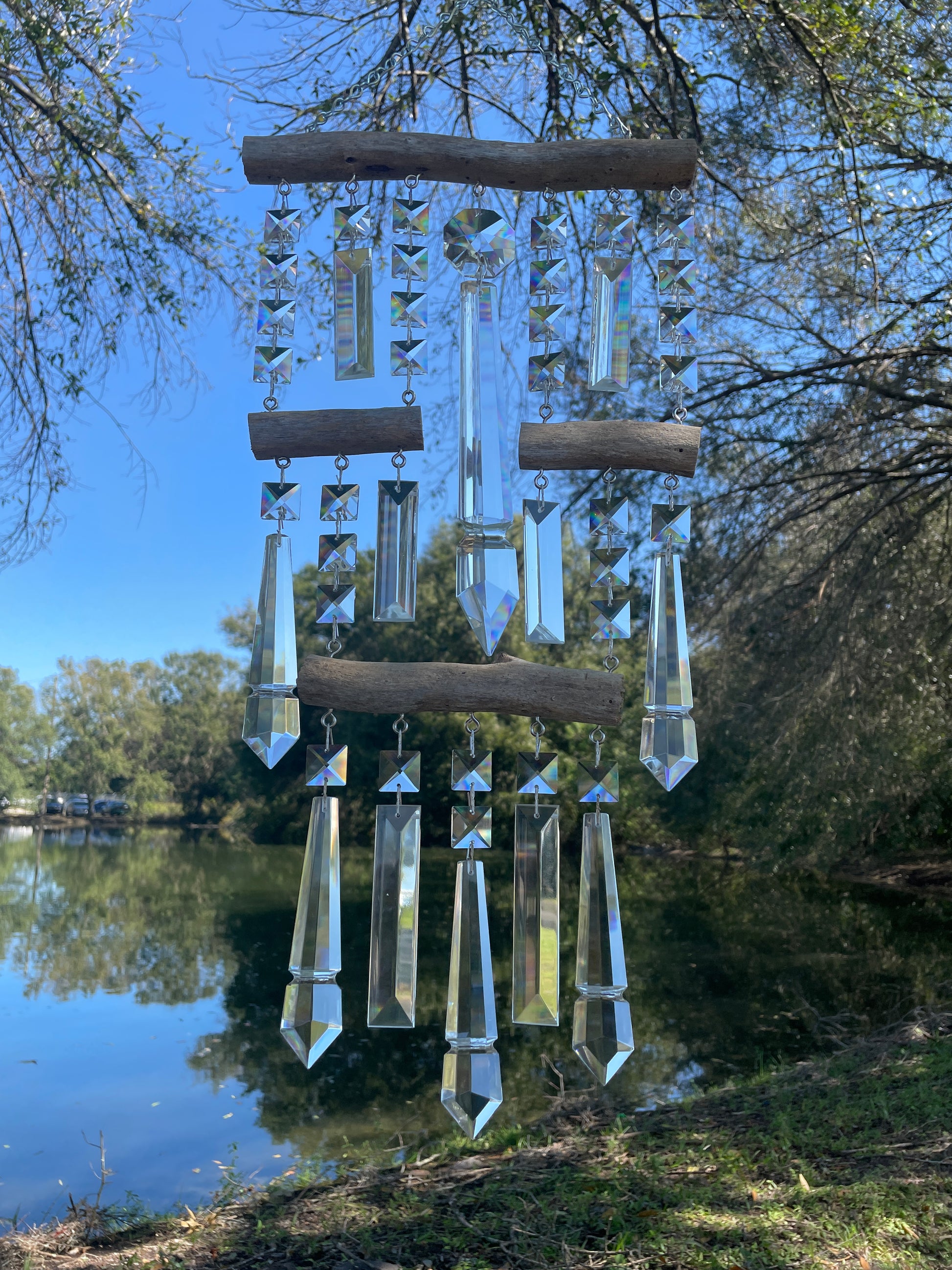This photograph features an intricate crystal wind chime set against a tranquil natural backdrop. The wind chime is constructed with four wooden bars; a long top bar, two shorter center bars, and another long bottom bar, each interconnected by fish eye hooks and white string. The crystals suspended from the bars are shaped like tapered rectangles and triangles, resembling prisms or icicles. The larger bottom bar holds five crystal pieces, while the middle bars have two crystals each. The entire structure almost fills the frame of the image, emphasizing its elaborate design and clear, crystalline elements.

In the background, there is a serene scene showcasing a broad cyan blue sky and a reflective pond bordered by grass and moss. To the right, a prominent tree stands amid a line of trees encircling the pond. Hints of distant structures can be perceived, though they remain indistinct. The image, bathed in daylight, displays a harmonious palette of rustic browns and greens alongside the transparency of the crystal chimes, conveying a peaceful afternoon ambiance.